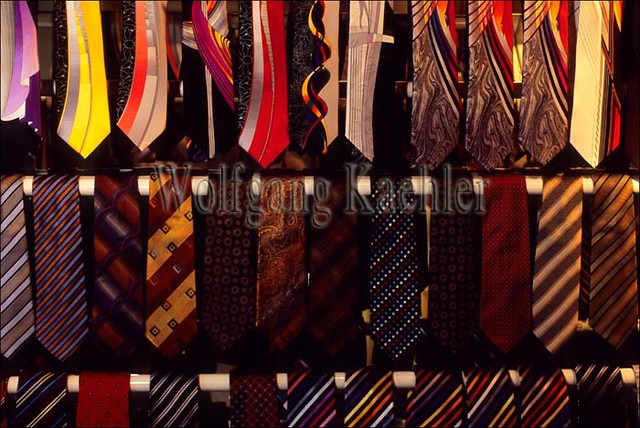The photograph features a close-up shot of three horizontal rows of neckties hanging over white rails, each tie looped over the rail and the short ends obscured from view. The middle row is fully visible, displaying a vivid array of designs and colors including diagonal stripes, multicolored patterns, and even sparkly or rhinestone embellishments. The top row is partially visible, with only the top portions of the ties extending out of the frame, showcasing some brighter and more exotic patterns. The bottom row is mostly cut off, revealing just the tops of the ties, yet it distinctly shows multicolored striped ties that match each other. Across the middle of the image is a translucent watermark with a black outline, reading "Wolfgang Kachler."